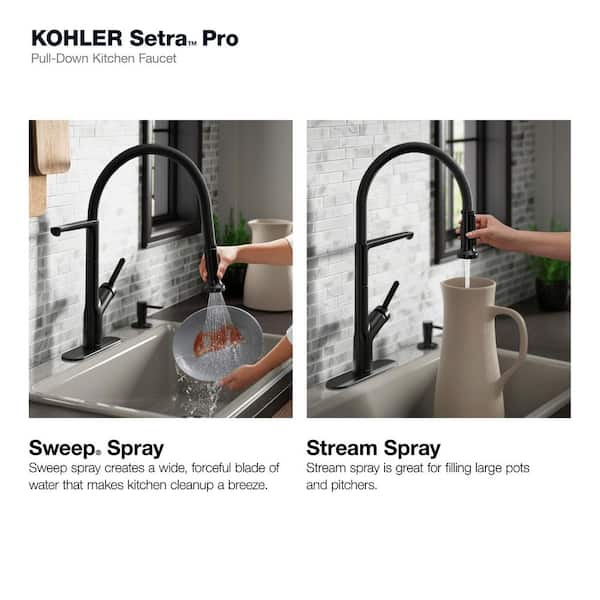The advertisement for the Kohler Setra Pro pull-down kitchen faucet features two side-by-side images showcasing the faucet in use. The title in dark black font reads "Kohler Setra™ Pro" with "pull-down kitchen faucet" in a lighter gray font below. The faucet itself is a large, arched, metallic black with a U-shaped handle.

In the first image on the left, a woman with white arms and hands uses the faucet's sweep spray mode to clean a blue plate with a red stain. This mode creates a wide, forceful blade of water, highlighted by the caption: "Sweep Spray creates a wide, forceful blade of water that makes kitchen clean-up a breeze." The background features a grey brick tiled backsplash and a clean, black countertop.

The second image on the right demonstrates the stream spray capability, where the same woman fills a beige pitcher. The caption reads: "Stream Spray is great for filling large pots and pitchers." The faucet is shown delivering a steady stream of water, perfect for such tasks. Both images highlight the practicality and versatility of the Kohler Setra Pro faucet in a modern kitchen setting.